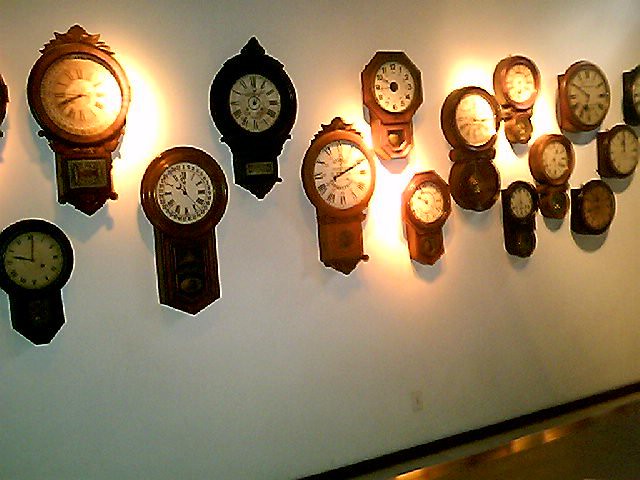The image depicts a collection of approximately 15 clocks adorning a white wall with black trim. Despite its low-quality resolution, the details of the clocks are discernible. The clocks extend horizontally from one end of the wall to the other, exhibiting various sizes yet maintaining a cohesive style. Some clocks feature standard numerals, while others display Roman numerals. 

The majority of the clocks are crafted from wood, presenting a range of shades from light to dark brown. Illumination is provided by three bright lights directed at the wall, highlighting the clocks. Certain clocks include plaques, likely indicating their branding, while others are equipped with tiny gongs or chimes. A few clocks are purely round, whereas most adhere to traditional wall clock designs.

The wall itself is stark white, interrupted only by a small electrical outlet near the lower center. The overall scene evokes a sense of rustic charm and nostalgia, enhanced by the dim quality of the image.